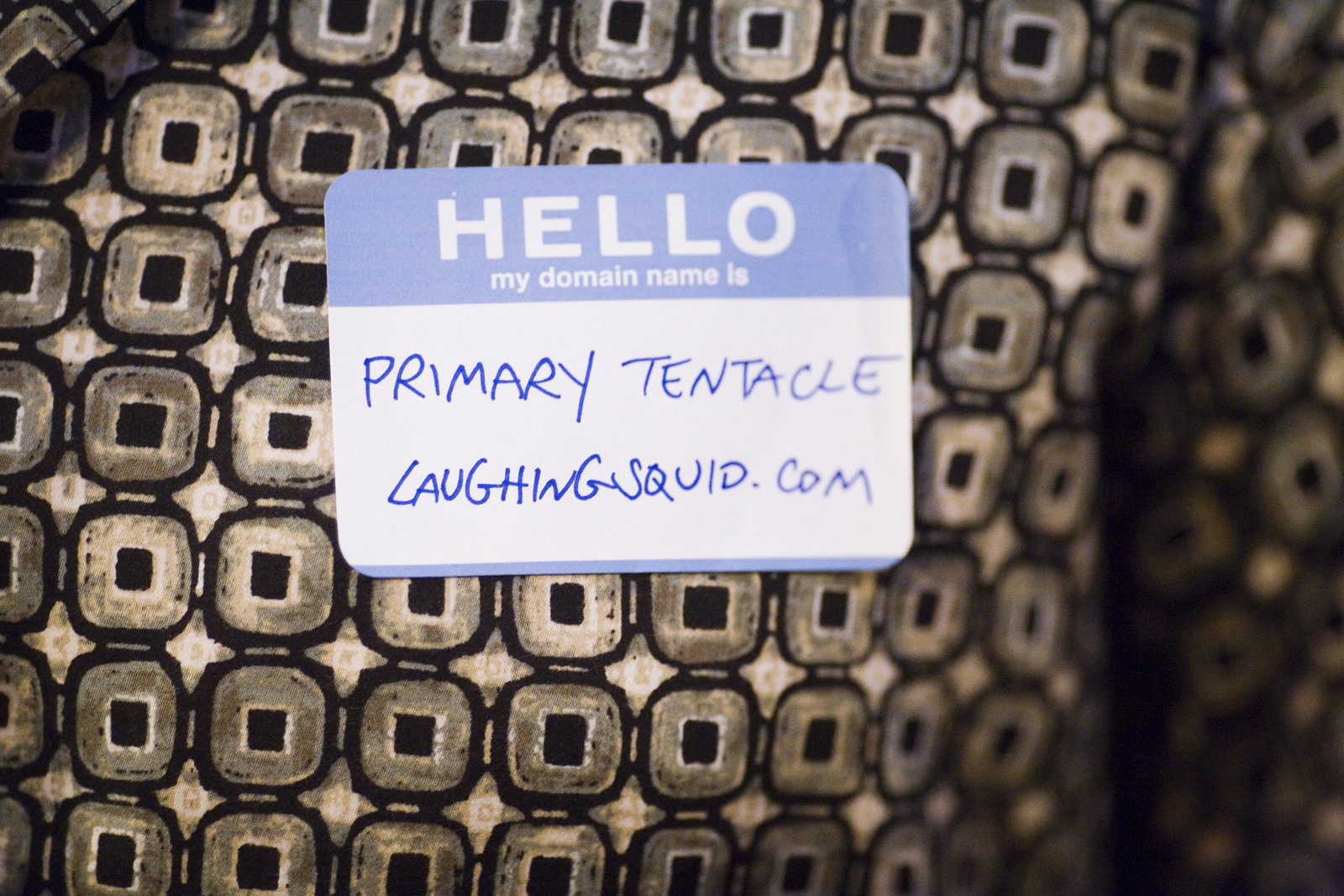The image depicts an extreme close-up of a textured surface resembling a shirt's chest area or possibly a tablecloth, featuring a distinctive pattern of rounded rectangles. These rectangles are outlined in black with a light brown inner fill and contain smaller squares that create a chain-link effect. Affixed to this patterned background is a rectangular name tag with rounded corners. The name tag has a blue header and footer, with the text "Hello my domain name is" in white. Below this, handwritten in blue pen, it reads "primary tentacle laughing squid.com" in all capital letters. The surface shows areas of shadowing, suggesting the photo was taken indoors. There is a faint water spot on the right side of the name tag, adding to the realistic texture of the image.